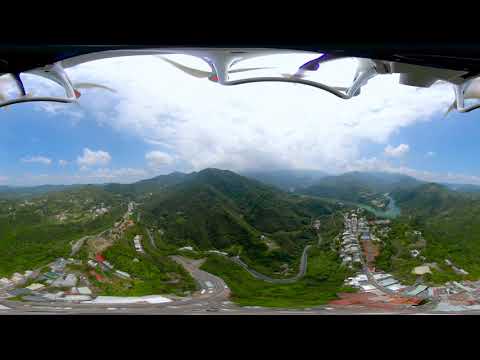The image features a top and bottom black border, framing an aerial view of a green, mountainous landscape interspersed with numerous paved roads and towns. Below the top black border, there are colored lines with hints of blue, red, and white, perhaps depicting a graphical overlay or map legend. The sky above the landscape is predominantly filled with massive white clouds, particularly in the center, while the right and left sides show clearer blue skies.

The terrain consists of densely green, sharp-pointed hills and mountains, with blacktop roads winding through them. These roads are accompanied by a series of buildings and infrastructure, lining the roads and nestled into the valleys. On the left and right of the image, towns and cities are visible, with a flowing body of water located above the town to the right. The overall geometry of the image appears slightly distorted, suggesting a wide-angle or panoramic lens was used.

Overall, the scene captures a detailed and vibrant view of a lush, well-developed area set against a dynamic sky, likely photographed during midday.